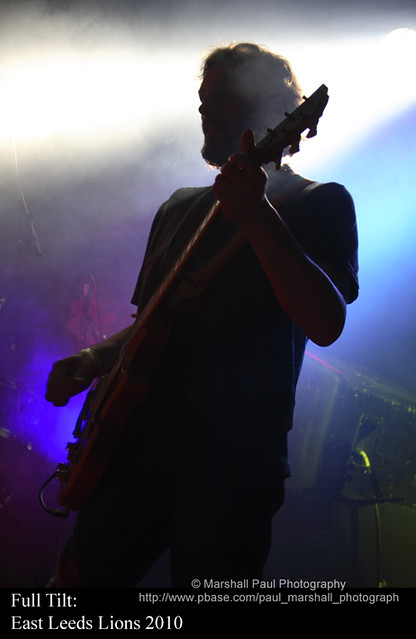The image is a striking photograph of a man playing a guitar on stage during a concert, heavily shadowed due to strong backlighting. The powerful lights behind him create a dramatic effect, rendering the front of his body and face mostly as a silhouette. Despite the shadows, it's evident that he is a white man with dark brown, tousled hair and a slight beard or goatee. He is wearing a dark t-shirt and pants, and there's possibly a bracelet or watch on his right wrist. The guitar he is playing has hints of red tone, partially illuminated by the stage lights. Surrounding him are beams of blue light and visible wisps of smoke, adding to the dramatic atmosphere. In the background, faint outlines of cases can be seen. Notably, the bottom left corner of the image has text that reads "Full Tilt East Leeds Lions 2010," while the right side is marked with "Marshall Paul Photography," suggesting the photographer's credit.